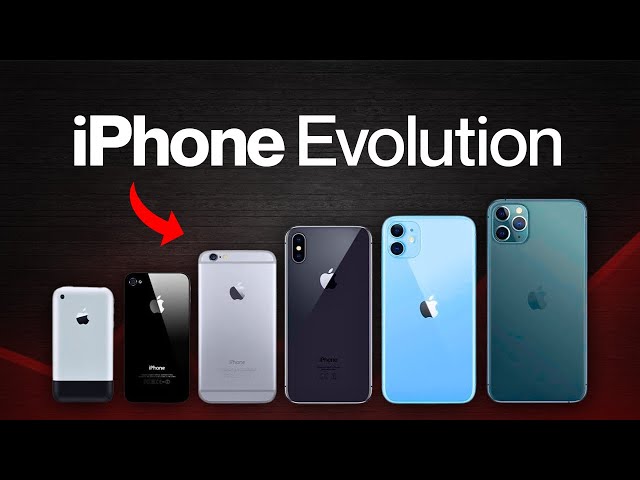The image showcases the evolution of iPhones over time with the title "iPhone Evolution" prominently displayed at the top in black text, accompanied by the Apple logo. From left to right, the image presents six successive generations of iPhones, each standing upright with the Apple logo visible, progressing from the smallest and simplest to the largest and most advanced. 

The first iPhone on the left is white with a black bottom section, followed by a black iPhone, a silver iPhone, a charcoal gray iPhone, a baby blue iPhone, and finally the largest, which is a teal-colored iPhone. The phones also vary in camera configurations: the first three models feature a single camera, the fourth and fifth models have two cameras, and the latest model on the far right boasts three cameras. The shiny finish on each device suggests they are being showcased in a well-lit setting, emphasizing the advancements in design and technology over the years. An arrow beneath the text points to the iPhone in the center, drawing attention to the progression in size, color, and camera capabilities, effectively illustrating the development of iPhones from their inception to the present day.